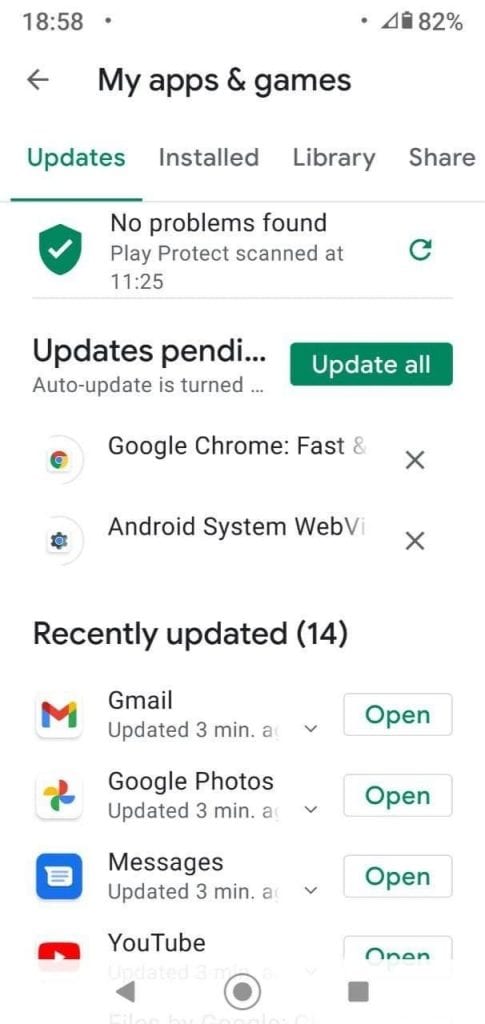The image is a screenshot from a mobile device, displaying a section of the Google Play Store interface with a white background and black text. 

In the upper left corner, it indicates the time as 18:58. To the right, a battery icon shows 82% charge remaining.

Centered below the status bar, there's a heading titled "My Apps and Games." Beneath this, a navigation bar features options for "Updates," "Installed," "Library," and "Share," with the "Updates" tab highlighted in green.

Below the navigation bar, a green shield icon with a check mark signifies "No Problems Found," accompanied by the text “Play Protect scanned at 11:25” and a refresh icon to its right.

A dividing line separates this section from the next, which begins with the heading "Updates Pending." To the right of this heading is a green "Update All" button. Two downloadable apps are listed beneath, each with an "X" icon to dismiss:
1. Google Chrome (marked as "Fast") 
2. Android System WebView

Further down, the heading "Recently Updated" is shown with the number 14 in parentheses. Four recently updated apps are displayed below, each with an "Open" button to the right:
1. Gmail - Updated three minutes ago
2. Google Photos - Updated three minutes ago
3. Messages - Updated three minutes ago
4. YouTube - Updated three minutes ago

This detailed view captures the state of app updates and security checks on the user's device at a specific time.